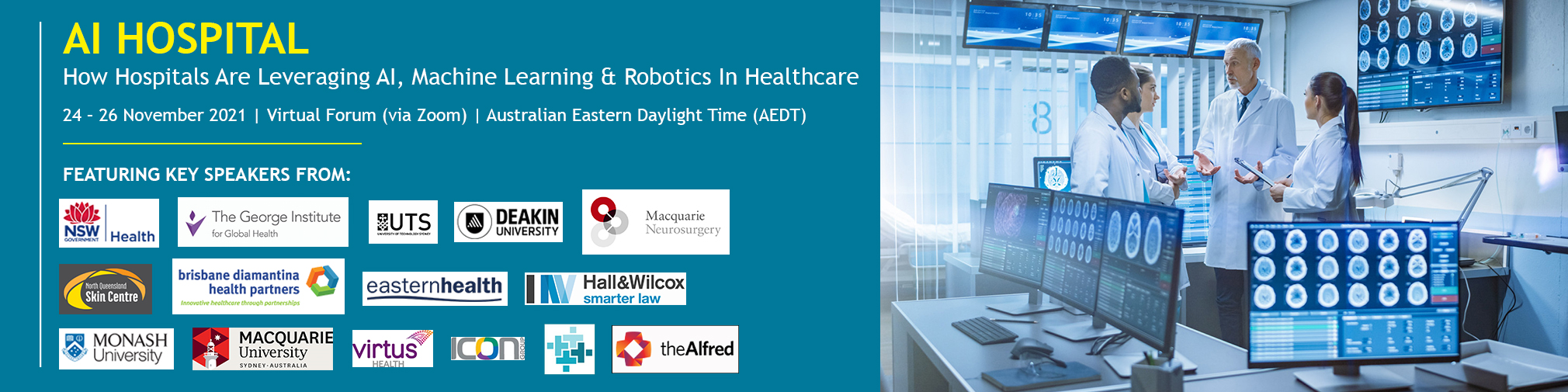**Detailed Caption:**

This image is a screenshot of an infographic promoting a virtual forum titled "AI Hospital," prominently displayed in yellow letters against a teal backdrop with white text. The event aims to discuss how hospitals are leveraging artificial intelligence, machine learning, and robotics in healthcare. Scheduled to take place from November 24th to 26th, 2021, the forum will be held virtually via Zoom, adhering to Australian Eastern Daylight Time (AEDT).

The screenshot also includes a photograph featuring four doctors in a laboratory environment, surrounded by multiple laptops. The doctors depicted are diverse: an older white male doctor, a black male doctor, and two female doctors. 

The infographic lists key speakers from various esteemed institutions and organizations, including NSW Health, the George Institute for Global Health, the University of Technology Sydney (UTS), Deakin University, Macquarie Neurosurgery, North Queensland Skin Center, Brisbane Diamantina Health Partners, Eastern Health, Hall and Wilcox Smarter Law, Monash University, Macquarie University, Virtus, Icon, and The Alfred. A distinctive logo in blue and teal with scattered dots, likely representing a sponsor or partner, is also visible.